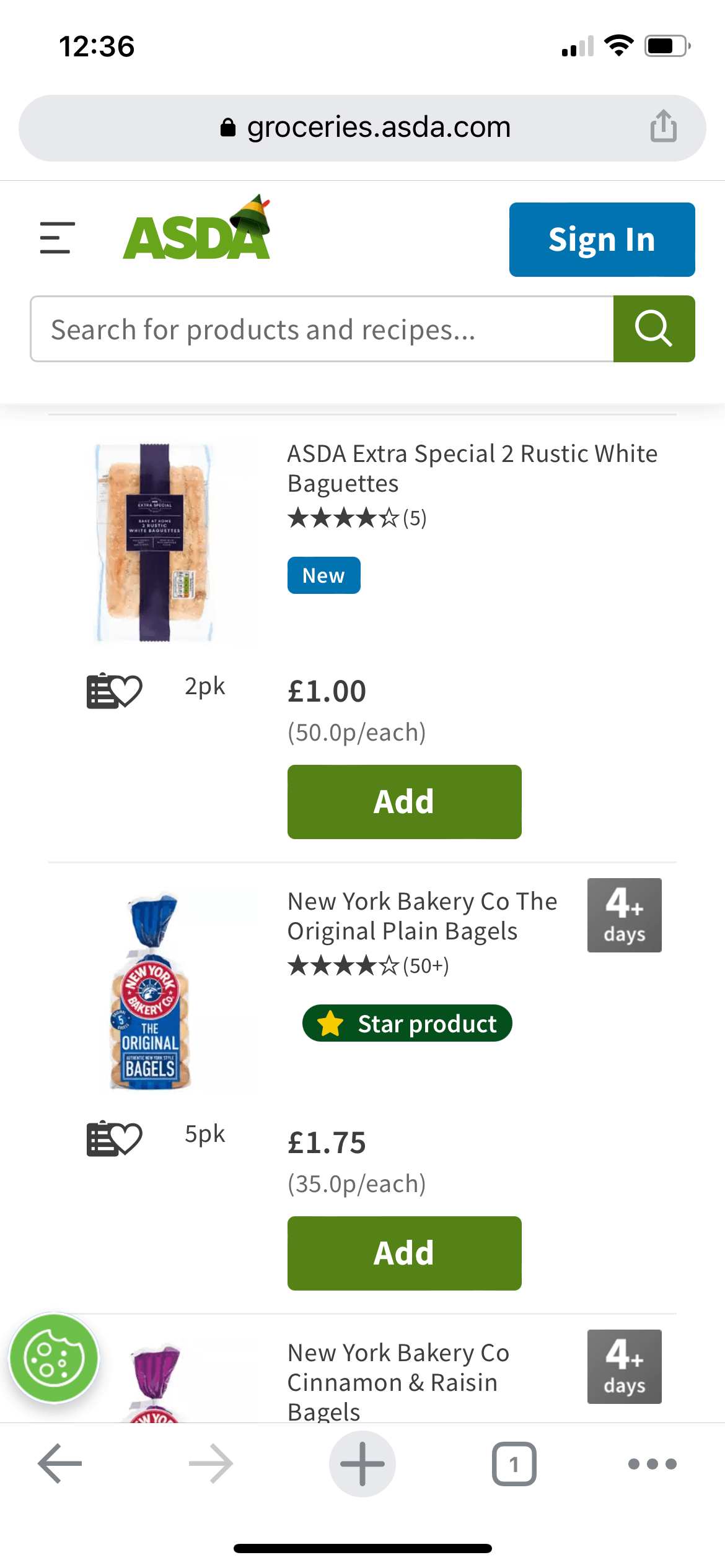The image is a screenshot from a mobile phone displaying a webpage, specifically from the ASDA grocery shopping site, groceries.asda.com. The phone's status bar at the top shows that the battery is about three-fourths charged, along with connectivity bars.

Below the status bar, in bold green capital letters, "ASDA" is prominently displayed with a distinctive hat or accent on the final "A". To the right of this logo is a blue "Sign In" button.

The screenshot also highlights a search area labeled "Search for products and recipes," accompanied by a green square with a white magnifying glass icon for executing the search.

Further down the page, the user has viewed specific grocery items:
1. "ASDA Extra Special Two Rustic White Baguettes," marked as a new product with options to add to the cart, click "Love," or add to a list.
2. "New York Bakery Company Original Plain Bagels," with an option to add to the cart.
3. "New York Bakery Company Cinnamon and Raisin Bagels," also available to add to the cart.

All listed products mention a freshness guarantee of "4+ days."